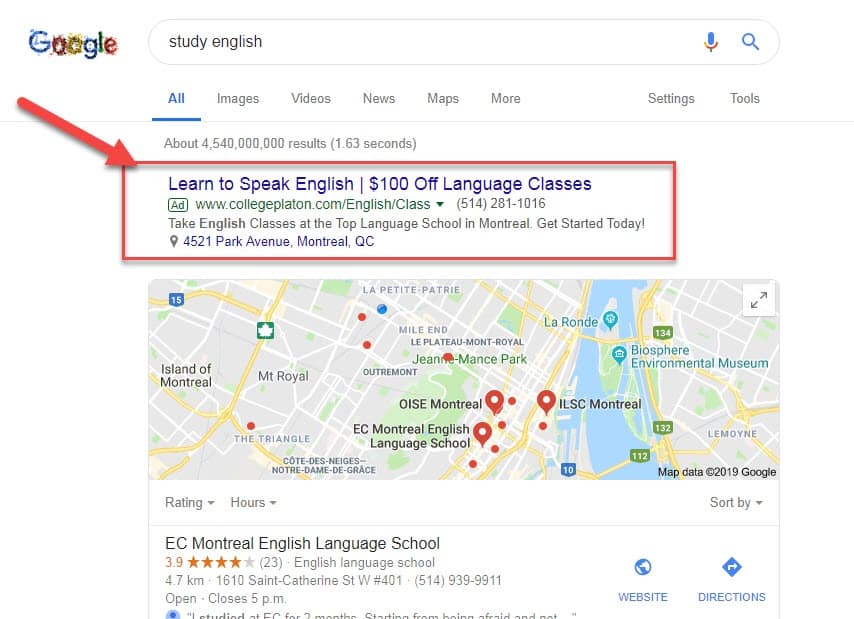In this image, a Google search results page is displayed with Google's festive colors, including elements reminiscent of holiday lights. The search query “study English” is typed in the search box, accompanied by a colorful microphone icon and a blue magnifying glass icon.

At the top of the search results, there is an advertisement highlighted with a red box and a red arrow pointing to it. The ad reads: "Learn to speak English - $100 off language classes." It indicates that it is a paid advertisement from the website collegeflayton.com, with further details provided including the phone number 514-281-1016. The text encourages potential students to "Take English classes at the top language school in Montreal" and to "Get started today". The address listed is 4521 Park Avenue, Montreal, Quebec. A small map within the image highlights various locations with red pinpoints. The advertisement also includes a rating and the hours of operation.

Beneath the advertisement, there is a listing for "EC Montreal English Language School," which has a rating of 3.9 stars out of 5, with 23 reviews. Four of the five stars are displayed in gold. The school is categorized as an “English language school” and is located 4.7 kilometers away, at 1610 St. Catherine Street West, number 401. The contact number for this school is 514-939-9911. The listing indicates the school is currently open and will close at 5 p.m., and it includes links for the website and directions.

Overall, the background is predominantly white, with the map section being colorful and displaying several pinpoint markers.